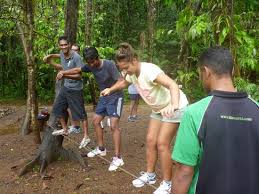This detailed photograph showcases a group of four people engaging in a balance activity in an outdoor jungle setting. The scene is characterized by a dirt clearing surrounded by dense, lush tropical foliage, including palm-like plants. In the center, a low rope or stick, close to the ground, runs horizontally across the frame, tied between two trees. The people, consisting of three men and one woman, are in a straight line and seem focused on balancing on this low-hanging rope. Each person is bent over with arms outstretched, emphasizing the difficulty and concentration required for this task.

On the far left, the woman is seen wearing white sneakers, light gray shorts, and a yellow or tie-dye t-shirt, with her hair tied up. Next to her, one man wears a dark-colored shirt and blue shorts, while another man beside him is dressed in a gray t-shirt and longer cargo-style shorts. The fourth individual, standing slightly apart and smiling, wears a gray t-shirt with shorter blue shorts. All participants are sporting white athletic shoes.

In the foreground, partially turned away from the camera, is a man acting as a coach or referee. He wears a black jersey with green sleeves and watches the group's feet intently. His posture suggests he might be overseeing the activity or perhaps guiding the participants. The image captures a moment brimming with focus and camaraderie, set against the vibrant backdrop of a jungle forest.